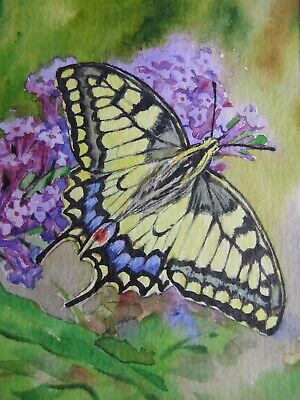This mixed media artwork features a highly detailed yellow butterfly as its focal point, delicately rendered with a combination of ink and colored pencils, displaying fine shading characteristic of colored pencils. The butterfly's wings are outlined in black and adorned with vertical black lines. A notable blue stripe runs along the bottom center of the wings, which culminates in two small tails, and a striking red dot is prominently visible at the bottom center of the wings. The butterfly, which has a furry-looking grey body, is perched atop a cluster of light purple flowers, surrounded by green foliage depicted in watercolor. The background consists of a green wash, giving an impressionistic, slightly faded look. This could be due to the age of the painting or an intentional effect suggesting an outdoor scene transitioning into evening. The background's less detailed, watercolor technique contrasts with the sharply defined butterfly, enhancing its prominence in the composition.